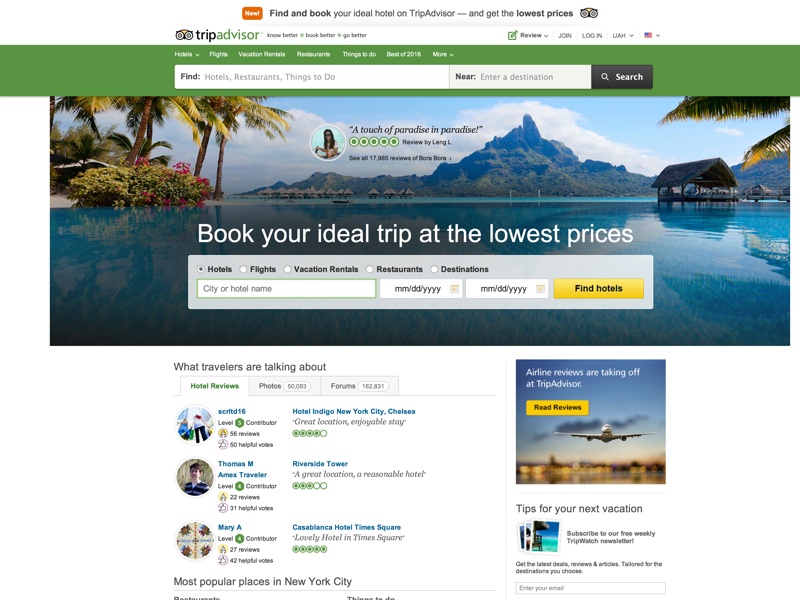Screenshot of the TripAdvisor homepage featuring a detailed layout. The top section includes the TripAdvisor logo, with "Trip" in black and "Advisor" in green, accompanied by an emblem resembling a pair of goggles or owl eyes on the left. This header is set against a white background.

Below the header, there is a prominent green bar housing the main search functionality, which is divided into two sections: "find hotels, restaurants, things to do" and "near enter destination." The search button on the right side of this bar is black with a white magnifying glass icon.

Further down the page, a vibrant banner image depicts a lush tropical beach with clear blue waters and an island in the distance, creating an inviting visual of an exotic destination.

In the lower portion of the screenshot, the layout showcases recent comments and reviews situated on the bottom left, providing users with authentic feedback and experiences from other travelers.